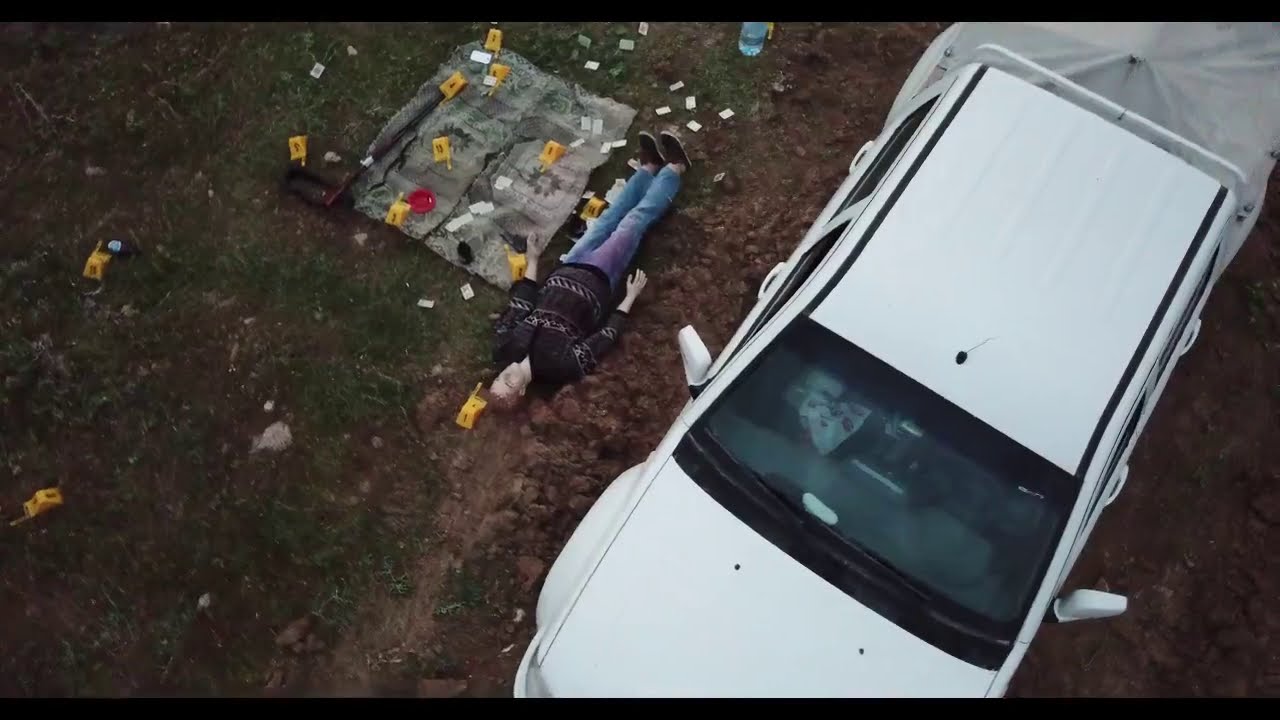The aerial photograph captures a staged outdoor crime scene featuring a white vehicle, possibly a van or SUV, situated on brown, soil-covered ground. To the left of the vehicle lies a mannequin, positioned flat on its back with legs extended, donning a black long-sleeve jersey, blue jeans, and black shoes. The mannequin's hands and head are stiff and unnaturally white, with a red stain on the upper right section of the jeans. Beside the mannequin is a dirty white sheet resembling a picnic blanket. Scattered around the sheet and mannequin are numerous yellow and white evidence markers, each labeled with numbers, emphasizing the staged nature of the scene. The setting includes a mix of green grassy areas and dirt around the mannequin and the vehicle, adding to the realism of the simulated crime scene.